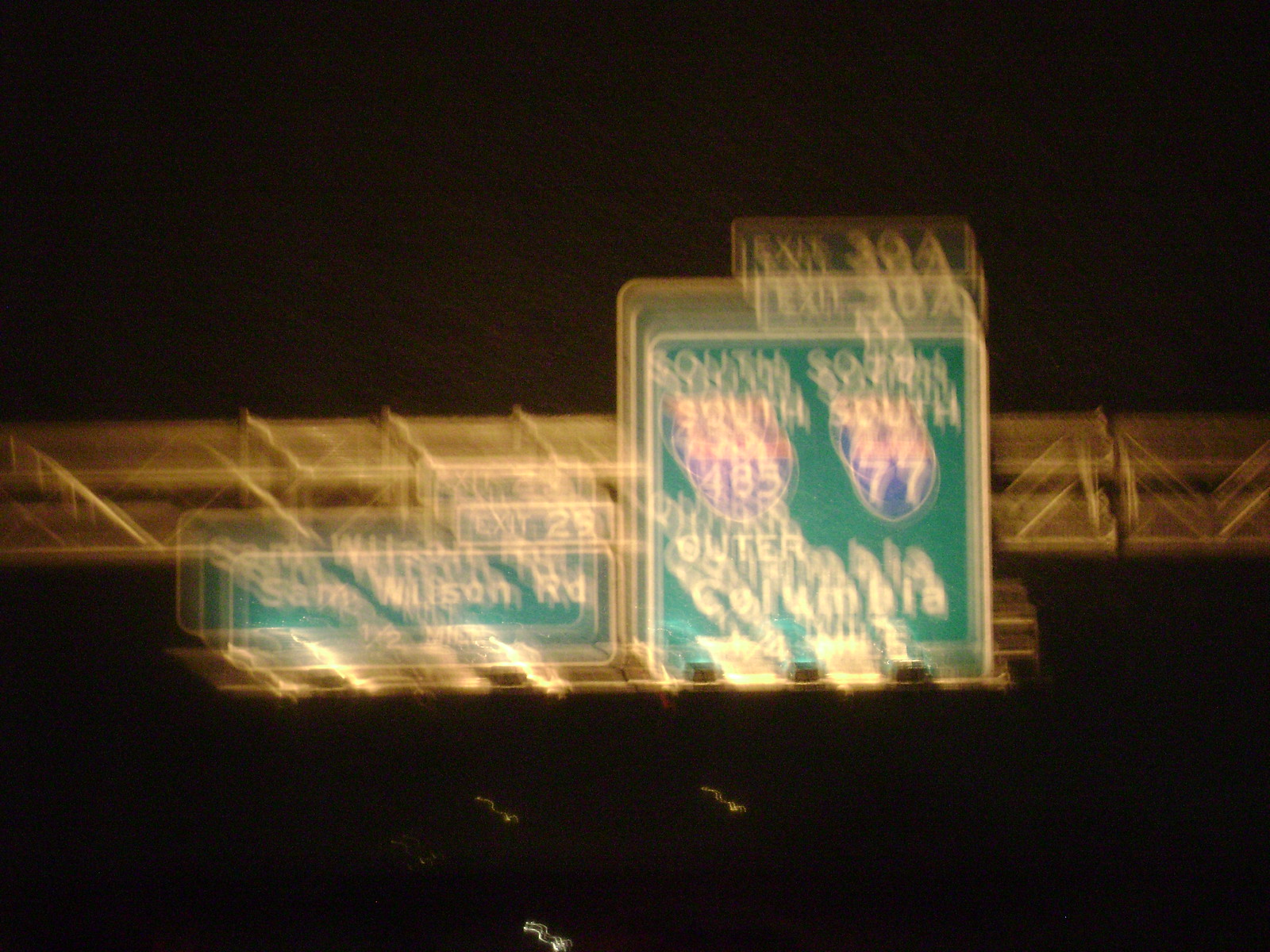A blurry photograph depicts an overhead highway structure displaying road signs. Although the image is not clear, the large green road sign features prominently, indicating directions for I-77 South and I-485 South, with I-485 also labeled "Outer." Additionally, the sign for "Sam Wilson Road, Exit 29" is visible. The indistinct lights in the frame suggest the presence of vehicles, hinting at nighttime or low-light conditions. The photograph appears to have been taken around Columbia, potentially South Carolina, given the familiarity of the location. Overall, the primary focus is the road sign mounted on the substantial overhead structure typical of interstates.